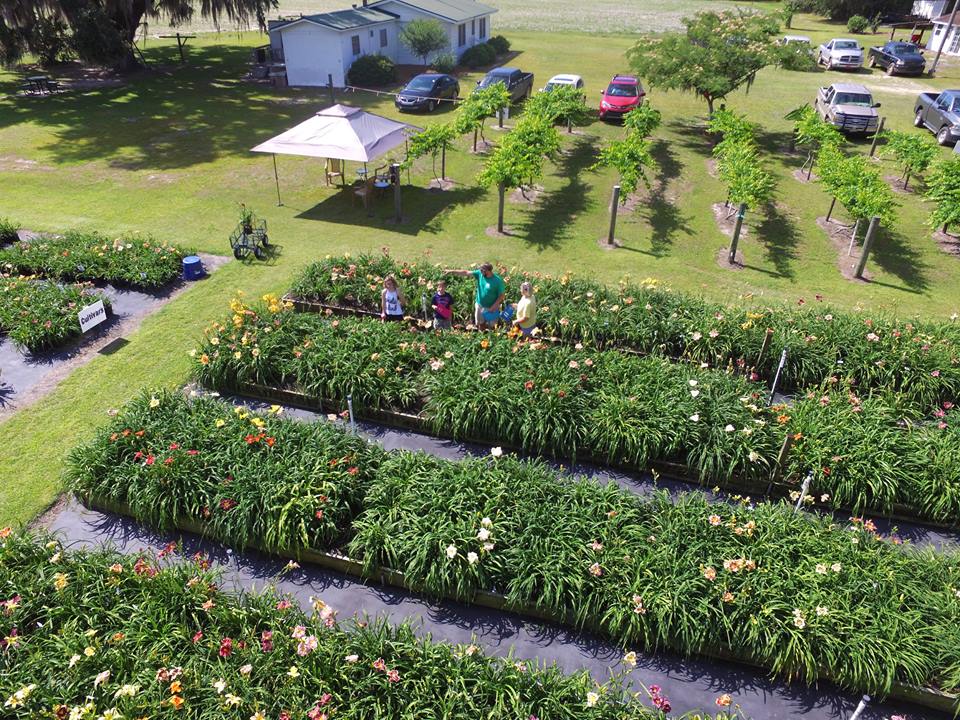The image showcases a vibrant garden center or nursery captured from an aerial or elevated perspective, possibly by a drone. The scene is bathed in bright sunlight, highlighting the meticulously organized rows of ornamental and flowering plants that are on sale. Interspersed among the rows of plants, a family comprising an adult, likely a mom, and three children can be seen carefully inspecting the flowers, which boast a vivid array of colors including yellow, pink, red, white, beige, and orange. Small trees are also visible, suggestive of being available for purchase. Toward the background, a small parking lot adjacent to a white house and a canopy is visible, with nine cars of varying colors like red, black, white, and beige-silver parked. A small shed is also seen on the left-hand side, complementing the overall pastoral and serene setting. The predominant colors of green foliage and white structures dominate the scene, creating a warm and inviting atmosphere. There is no text in this image.